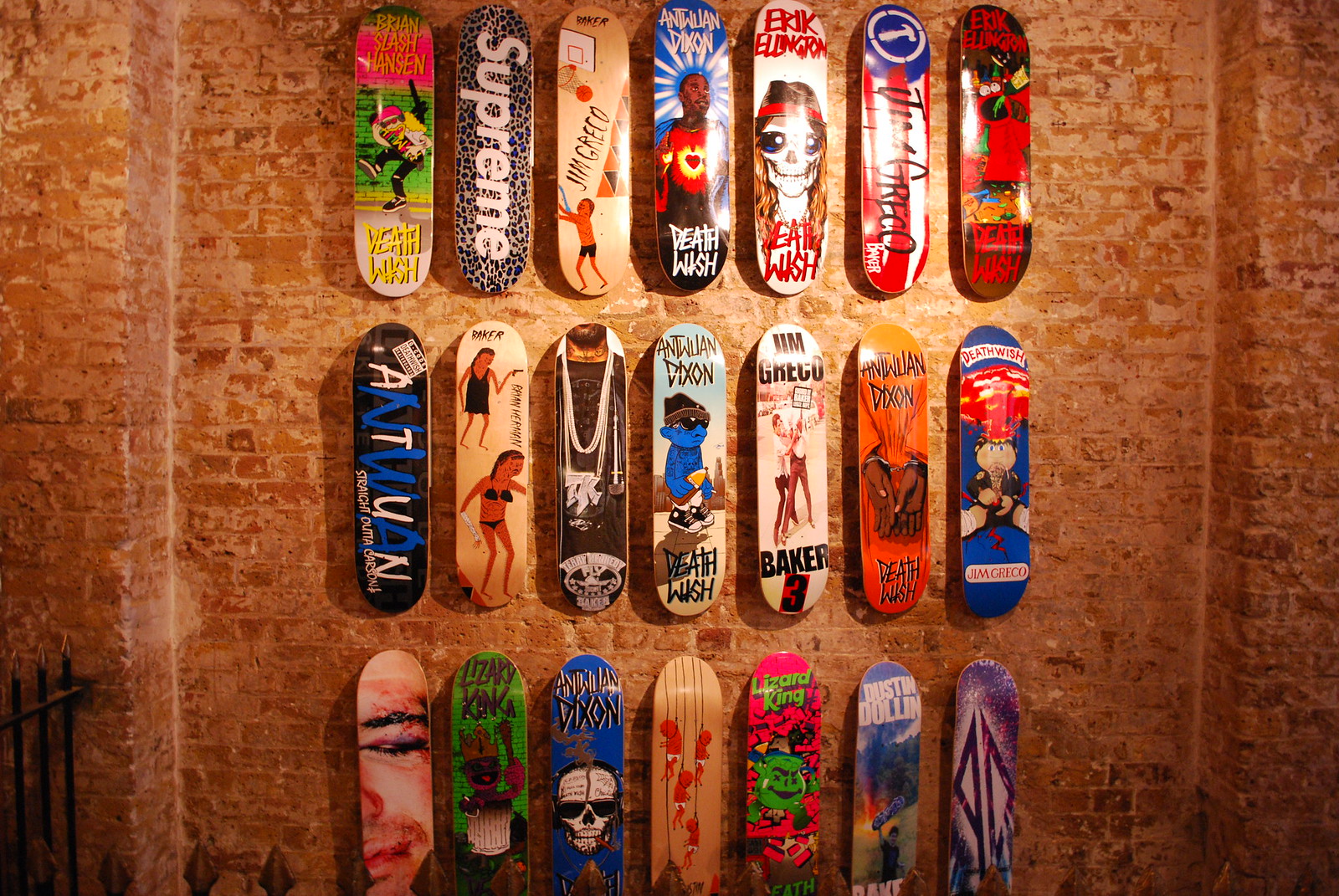The image depicts a colorful and vibrant collection of 21 skateboards hanging on a brown corkboard-type wall in a garage. Organized neatly into three rows of seven, each skateboard showcases the top side with a plethora of vivid designs and graphics. The color palette includes shades of red, blue, black, green, yellow, orange, purple, white, pink, and gold. Among the various graphic designs, some feature human forms, such as a girl in a bikini, faces, and skeletons, while others display brand names and text. Notable mentions include "Death Wish," "Supreme," "Baker," and possibly "Eric Ellinger" and "Jim Greco," although some text is too small to read. The diverse array of skateboards creates a striking visual with their intricate designs and bold colors against the faded brown backdrop.